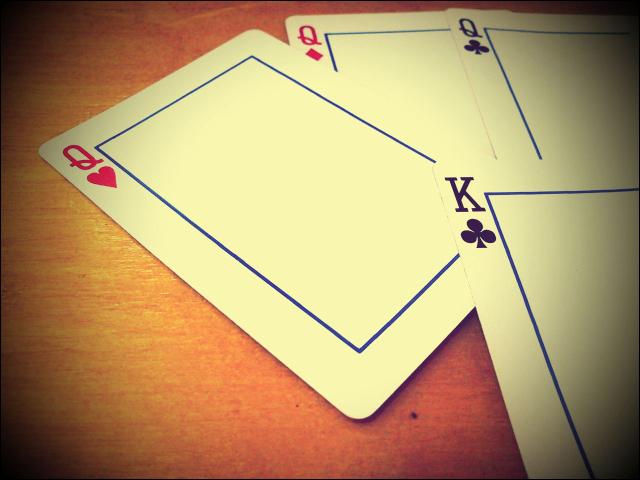In this photograph, four playing cards from a deck are elegantly displayed on a rustic wooden table. The edges of the image are subtly darkened with black highlights, focusing attention on the serene arrangement of the cards. Among them, three cards are neatly aligned side by side: the Queen of Hearts, the Queen of Diamonds, and the Queen of Clubs. Surmounting these three is the King of Clubs, positioned centrally on top. Notably, each card features a distinctive design—an empty square box bordered in black against a pristine white background. Unlike conventional playing cards, these unique designs lack the traditional illustrations of royalty, offering a minimalist and modern take on the classic deck.